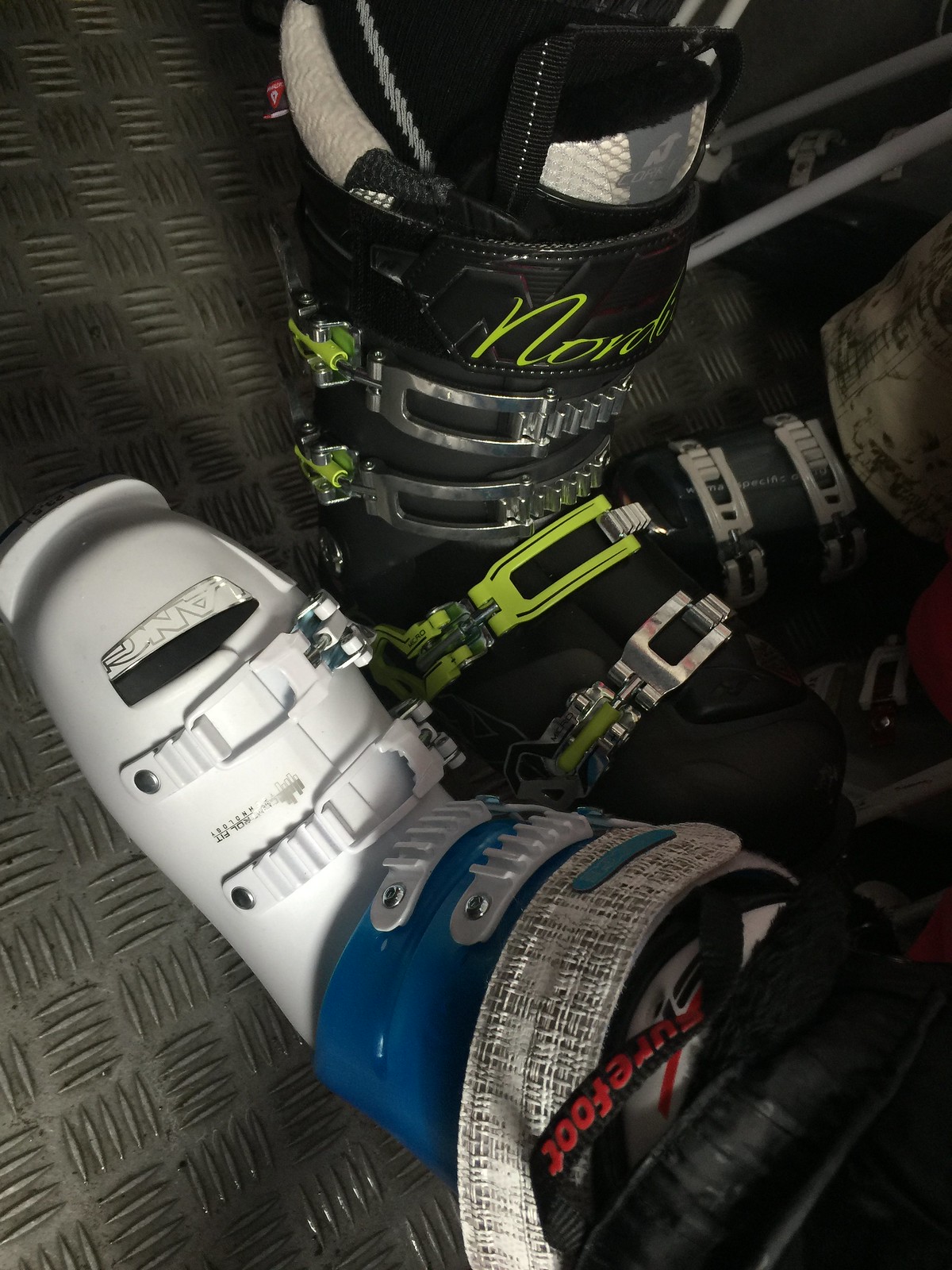This image showcases a set of ski boots, prominently featuring two boots side by side with a third boot lying to the right. The first boot is predominantly white with white buckles and a blue insulated vertical portion, equipped with a closure at the top to keep out snow. Directly beside it, the second boot is black, featuring silver closures and buckles along with a liner to prevent snow intrusion. A hint of neon green cursive font adorns the upper part of this black boot, though it’s partially obscured. The third boot, a dark one, is positioned on the far right of the image. These ski boots rest on a black rubber mat, distinguished by a textured pattern composed of squares and lines facing different directions. The background hints at two gray holes, adding to the gritty, industrial aesthetic of the scene.